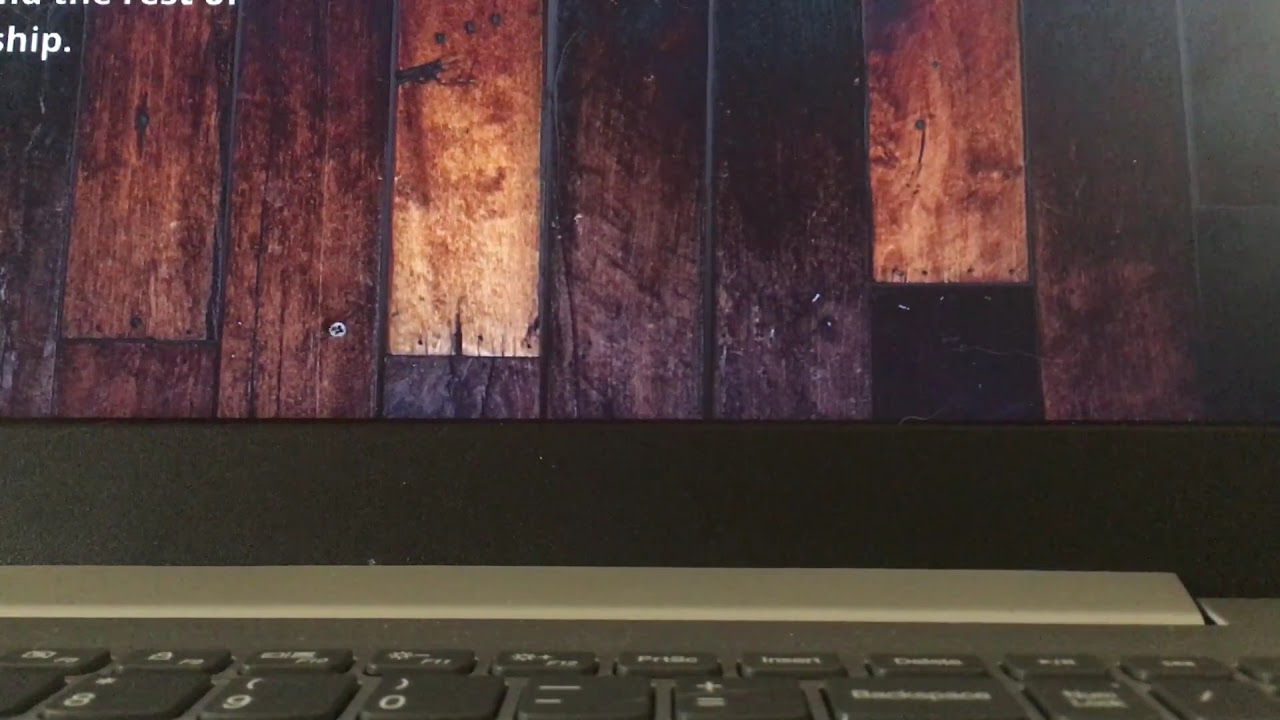This image features a close-up perspective of a laptop in landscape orientation, with the viewpoint starting from the keyboard. The lower part of the image showcases around the top half of the black keyboard, allowing visibility of keys such as the numeric keys (8, 9, 0) and various command keys, all featuring white text. Above the keyboard lies the silver hinge that connects the keyboard to the screen.

The screen itself is bordered by a black bezel and displays a high-resolution close-up image of narrow wood boards arranged vertically. These wood boards vary significantly in color, ranging from light to dark shades of brown. In the upper left-hand corner of the screen, partial text is visible, ending with the letters "H-I-P-P-E-R-D." The photograph also highlights the textured, uneven coloring of the wood, suggesting a mix of different wood types.

Overall, the composition draws attention to the detailed craftsmanship of the wood on the screen and captures the sleek design elements of the laptop keyboard and hinge.